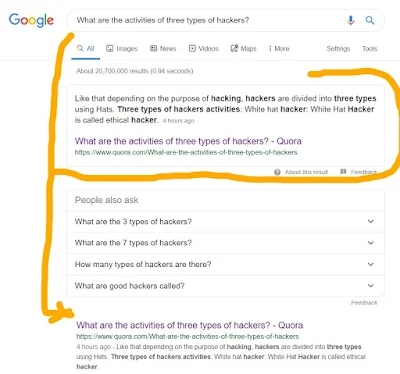This image depicts a Google search results page. At the upper left corner, the Google logo is prominently displayed. To the right of the logo is the search bar, where the query "what are the activities of three types of hackers" is entered. Just below the search bar, there is a horizontal menu offering options such as All, Images, News, Videos, Maps, More, Settings, and Tools.

Directly beneath the menu, the search results begin to appear. The first blurb starts with an introductory line mentioning the division of hackers into three types based on the purpose of hacking. This is followed by a brief explanation stating that hackers are categorized by different colored hats: white, gray, and black. The description for "White Hat Hacker" indicates that they are also known as ethical hackers.

Further down, the search results include multiple links. The first link title reads, "what are the activities of three types of hackers." The second link is a duplicate, also titled "what are the activities of three types of hackers," both leading to pages on the website Quora.